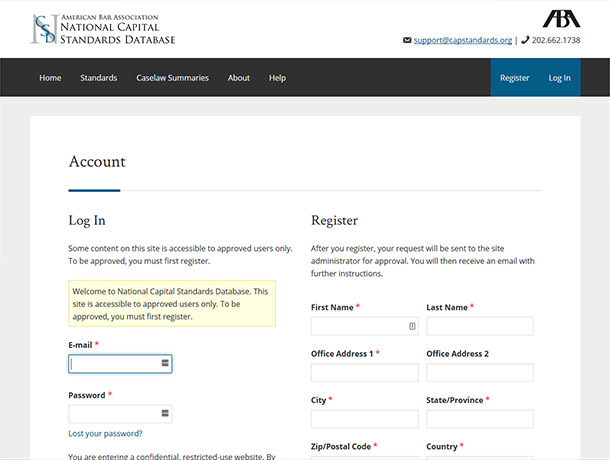Caption: 

"The sign-in page for the American Bar Association's National Capital Standards Database is displayed prominently. On the right side of the screen, a contact phone number is visible. The top navigation bar, set against a black background, includes tabs for 'Home,' 'Standards,' 'Case Law Summaries,' 'About,' and 'Help,' along with 'Register' and 'Login.' The 'Register' and 'Login' options stand out with a distinctive ACWA-colored background. The 'Account' section emphasizes that access to certain content requires approval and user registration. It provides fields for entering an email and password, with an option to recover a lost password. Below this, a notice highlights that visitors are entering a confidential, restricted-use website. On the right-hand side, the registration form seeks the user's name, office address, and country, indicating that site administrator approval is required after registration. The rest of the page beyond this point is not visible."